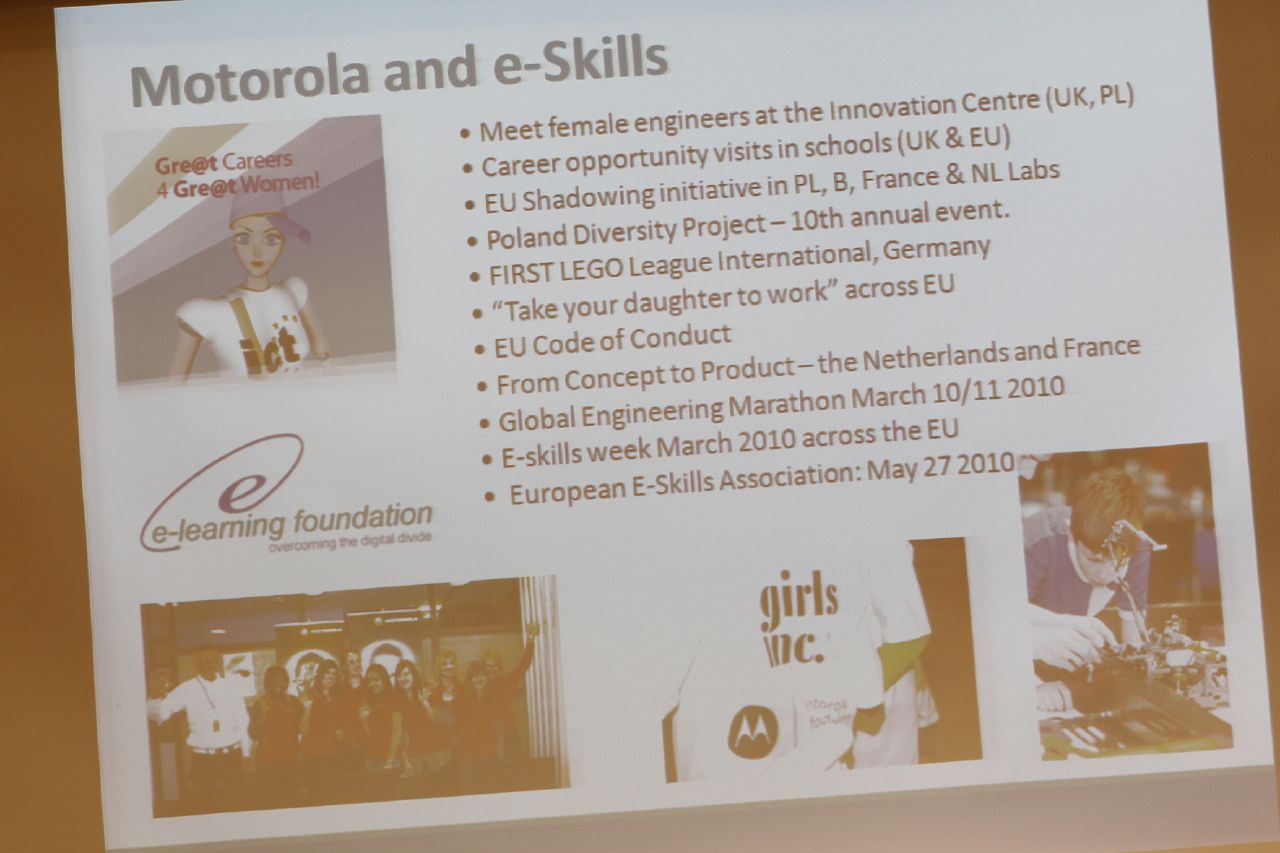This image appears to be a faded screenshot of a PowerPoint presentation slide, slightly rotated counterclockwise, with a white background and black text detailing initiatives by Motorola and eSkills. In the upper left-hand corner, the heading reads "Motorola and eSkills." Below this, there is a small square featuring an animated character of a woman or girl with blue hair or a blue cap, wearing a white t-shirt with red letters that read "ICT". Above this character, the text "Great Careers for Great Women" is prominently displayed. Adjacent to this image, a logo says "eLearning Foundation Overcoming the Digital Divide."

Dominating the middle and extending to the right of the slide are multiple bullet points detailing various initiatives and events, such as: "Meet female engineers at the Innovation Center (UK, PL)", "Career opportunity visits in schools (UK and EU)", and "EU shadowing initiatives in PLB, France, and NL labs". Other entries highlight events like the "Diversity Project 10th Annual Event", "First LEGO League International Germany", "Take Your Daughters to Work (EU)", "Code of Conduct from Concept to Product (Netherlands and France)", "Global Engineering Marathon (March 10-11, 2010)", "eSkills Week (March 2010 across the EU)", and the "European eSkills Association (May 27, 2010)".

At the bottom of the slide, stretching across the width, there is a series of photographs. The first image on the left shows a group of women standing together. The middle image features individuals wearing white t-shirts with the "Girls Inc." logo. On the far right, there is a picture of a young boy engaged with electronic devices or parts.